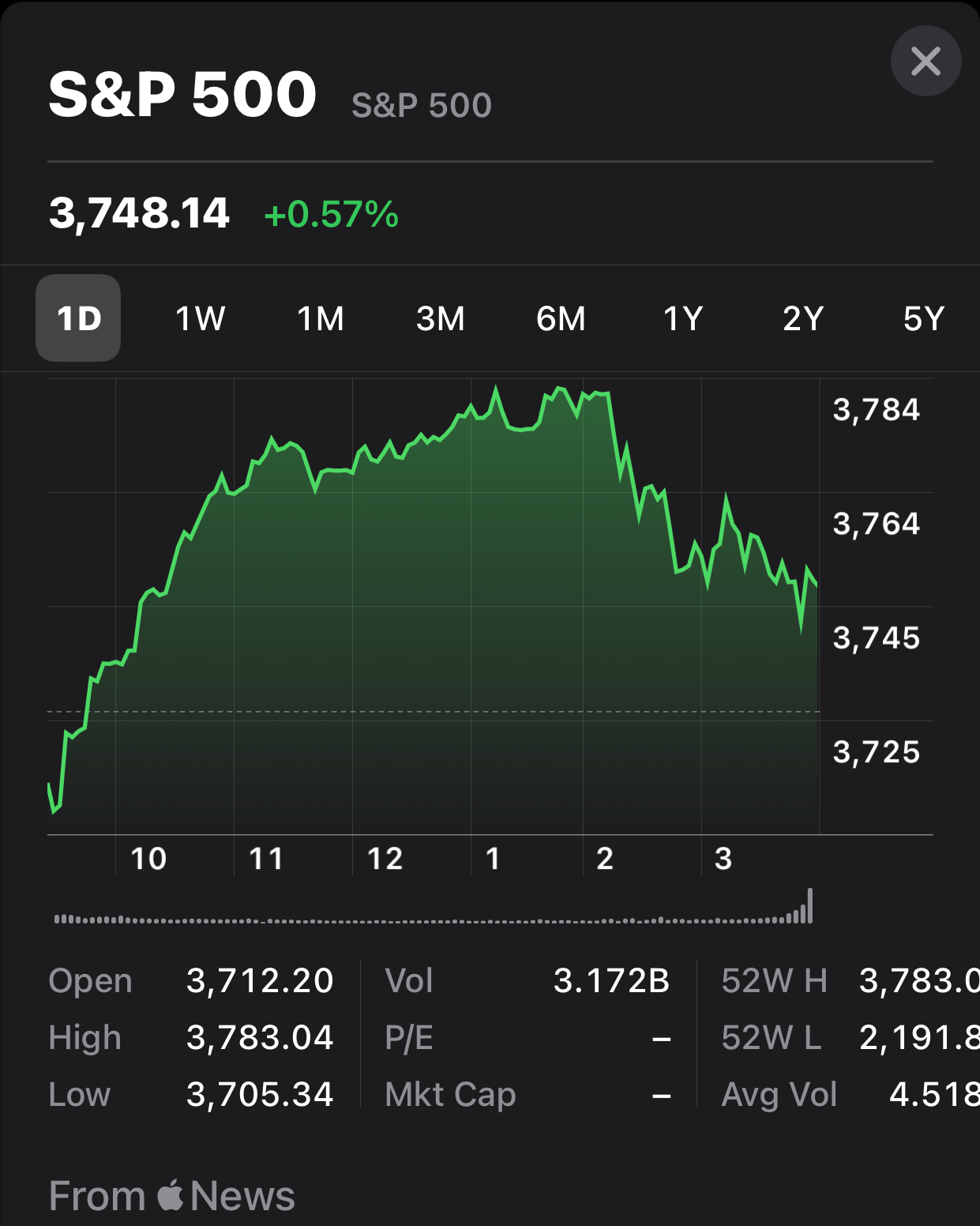This image captures a mobile screenshot of a stock chart financial information page, displayed on an app or website, with a distinctive black background. In the top-left corner, bold white letters spell out "S&P 500," accompanied by smaller gray text to its right repeating "S&P 500." In the top-right corner, there's a light gray circle containing a white 'X,' allowing the user to close the window.

Below this, a thin gray line serves as a border separator. The stock's current value is prominently shown in thick white numerals as "3,748.14," with a thinner green font indicating a positive change of " +0.57%." Another thin line separates this from the time frame options directly beneath it, which include "1D, 1W, 1M, 3M, 6M, 1Y, 2Y, 5Y," with the "1D" option highlighted by a gray box.

The main section shows the stock chart on a black background with light green gridlines forming squares. The price movements are displayed as a bright neon green line graph. Notably, the line peaks at the 6M mark, dips significantly over the one-year period, and continues to decline gradually thereafter. To the right, a column of gray-boxed numbers indicating price levels is shown, listing "3784, 3764, 3745, 3725" from top to bottom. The bottom axis features time markers labeled "10, 11, 12, 1, 2, 3."

Below the line chart is a small bar chart representing historical price movements, starting with flat, small rectangular bars that gradually increase in height towards the end. 

At the bottom of the image, detailed price information is listed in gray and white fonts. On the left:
- "Open" is 3712.20
- "High" is 3783.04
- "Low" is 3705.34

A thin vertical gray separator divides these from additional information to the right:
- "Val" is 3.172B
- "P/E" and "Market cap" show dashes (indicating missing data).

Further right, separated by another thin vertical line, are more price details:
- "52W H" (52-week high) is 3783.0 (cut off at the end)
- "52W L" (52-week low) is 2191.8
- "Avg Val" (average volume), partially visible, reads 4.518.

At the very bottom-left corner, a gray watermark contains the text "From" followed by an Apple icon and "News."